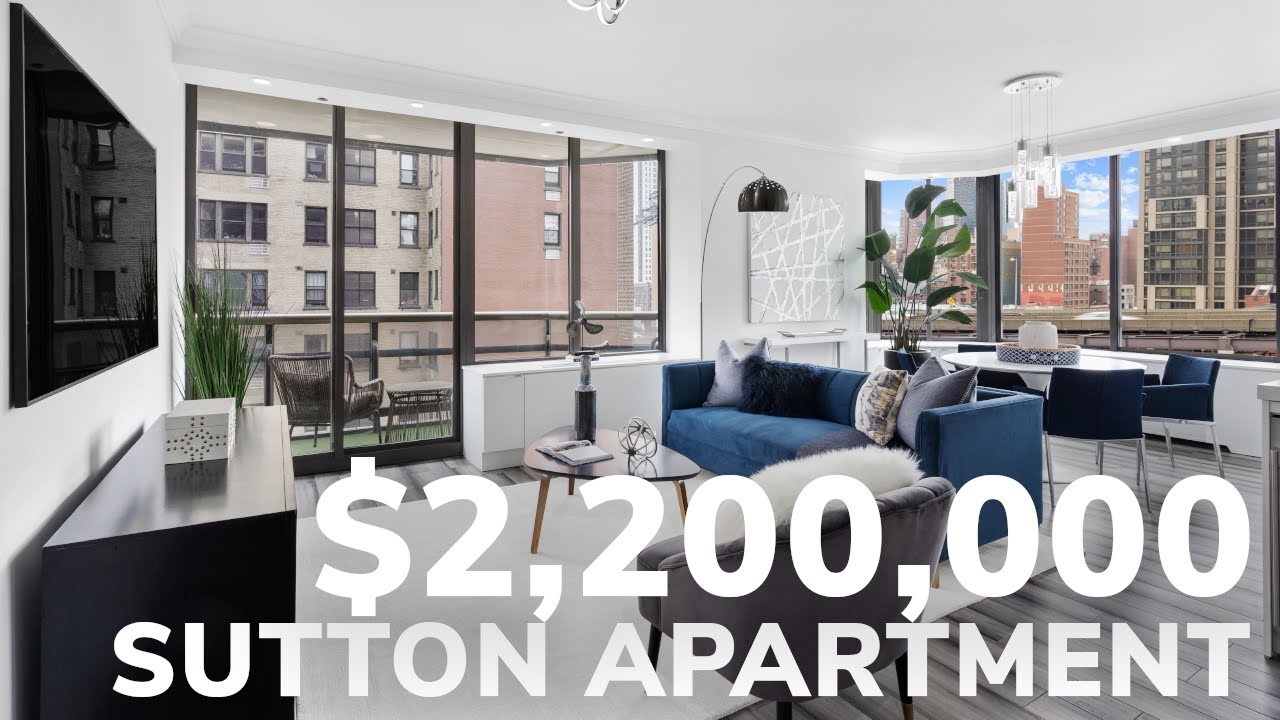This photograph, in a horizontal rectangle format, captures the interior of a modern apartment with vast windows on two walls, revealing other apartments nearby with floor-to-ceiling windows, and an outdoor balcony. The spacious living area features a stylish blue couch and a dining room table surrounded by matching blue upholstered chairs. Large, white, all-capitalized text stating "2,200,000" is prominently placed in the bottom right corner, extending nearly to the left side.

Mounted on one wall is a flat-screen TV, with a dark brown wooden console situated beneath it. The room is anchored by a white carpet on top of polished dark brown wooden floors. A vibrant green plant adds a touch of nature from the corner. The photograph highlights the luxurious feel of the apartment, reinforced by the price tag of $2.2 million, without any additional URLs or information.

Bright natural light floods the space, with a modern chandelier hanging over the dining area. The day appears sunny, dominated by a clear blue sky with a few white clouds, enhancing the overall ambiance of this sophisticated urban dwelling.